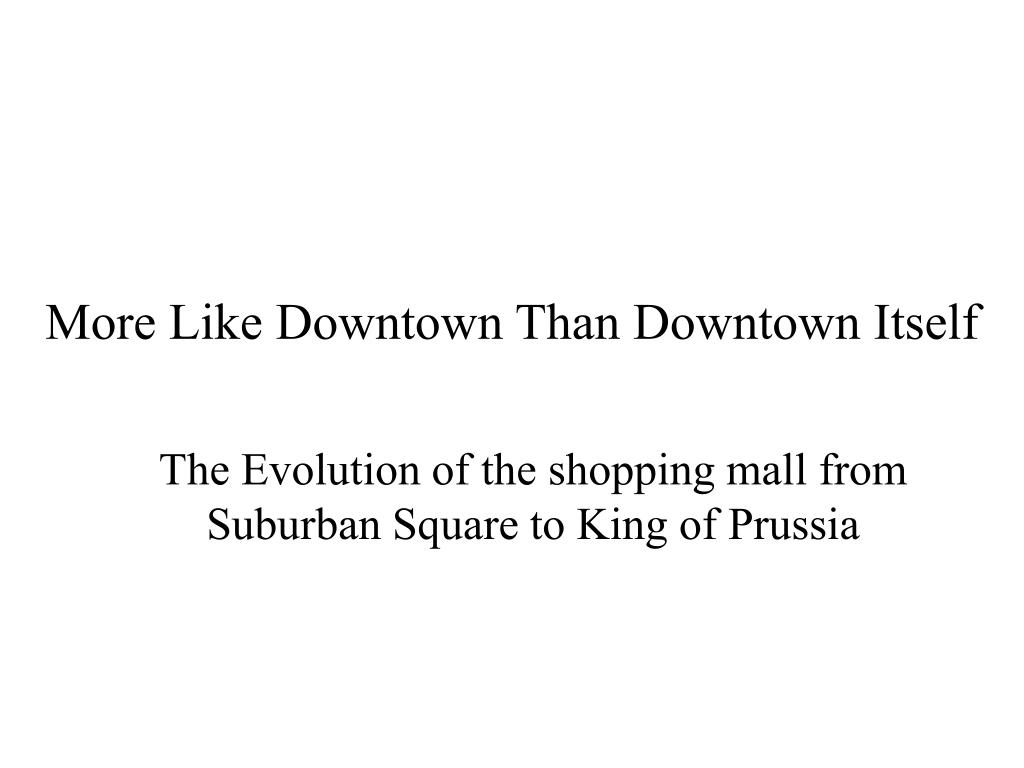The image is purely textual with a white background and black text. It resembles an advertisement or informational piece, likely for a presentation on the evolution of shopping malls. The content reads: "More like downtown than downtown itself" in a larger font at the top. Below this headline, in smaller font, are two lines that continue with, "The evolution of the shopping mall from suburban square to King of Prussia." The entire text sequence captures the progressive transformation of shopping malls, emphasizing a shift from generic suburban squares to notable destinations like King of Prussia.